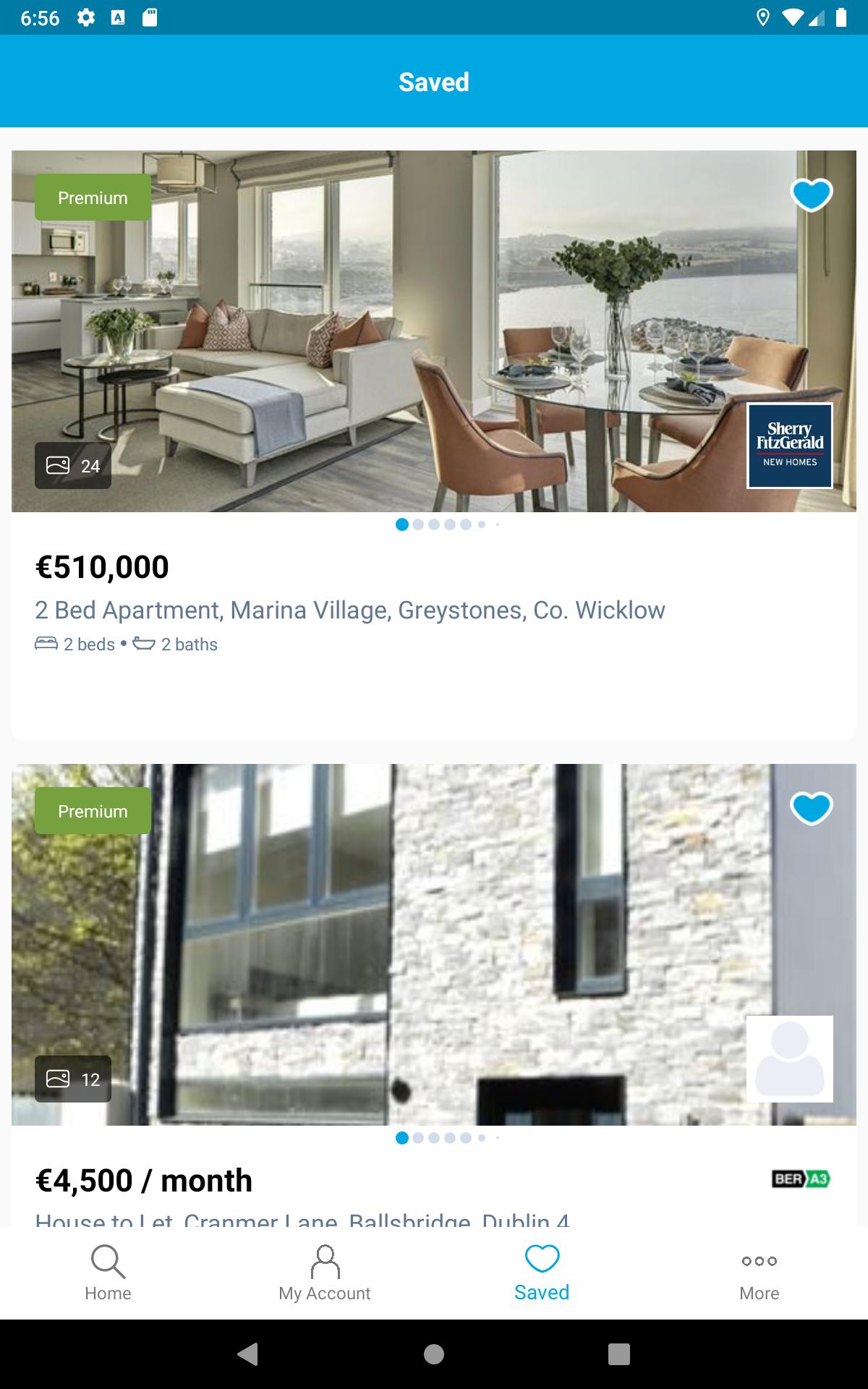A detailed snapshot of a cell phone screen capturing real estate listings. At the top-left corner, a darker blue box features white text displaying "656" beside a settings icon and a square box with the letter "A." Adjacent to them is an unidentifiable white box. The top-right corner shows a series of icons: a pin, Wi-Fi, a cellular signal (half strength), and a fully charged battery. Below this, a lighter blue rectangular box displays "Saved" in white text.

The first listing showcases a picturesque property—a house by a lake with mountains in the background. A green, square label with white text reading "Premium" is at the top-left of the image, while the top-right corner holds a blue heart icon with a white border. The image features a living room and a family room. The living room has an off-white couch with a blue towel draped over it. A glimpse of the kitchen reveals cabinets and an island. In the foreground, a round table is accompanied by pink chairs and adorned with flowers. Below this image, the text reads:

"£510,000, two-bedroom apartment, Marina Village, Gravestones, Commercio, Weekly."  
"Two beds, two baths."

The second listing advertises a rental property for £4,500 per month, showing only the building's exterior. It bears similar icons: a green "Premium" label at the top-left and a blue heart icon with a white border at the top-right. The text below the image states:

"£4,500 per month, House to let, Creamer Lane, Ballsbridge, Dublin 4."

At the bottom of the screen, navigation icons include a home button, a profile icon labeled "My Account," a "Saved" button highlighted in blue, and a "More" button. The footer is black with white icons—a left arrow, a circle, and a square.